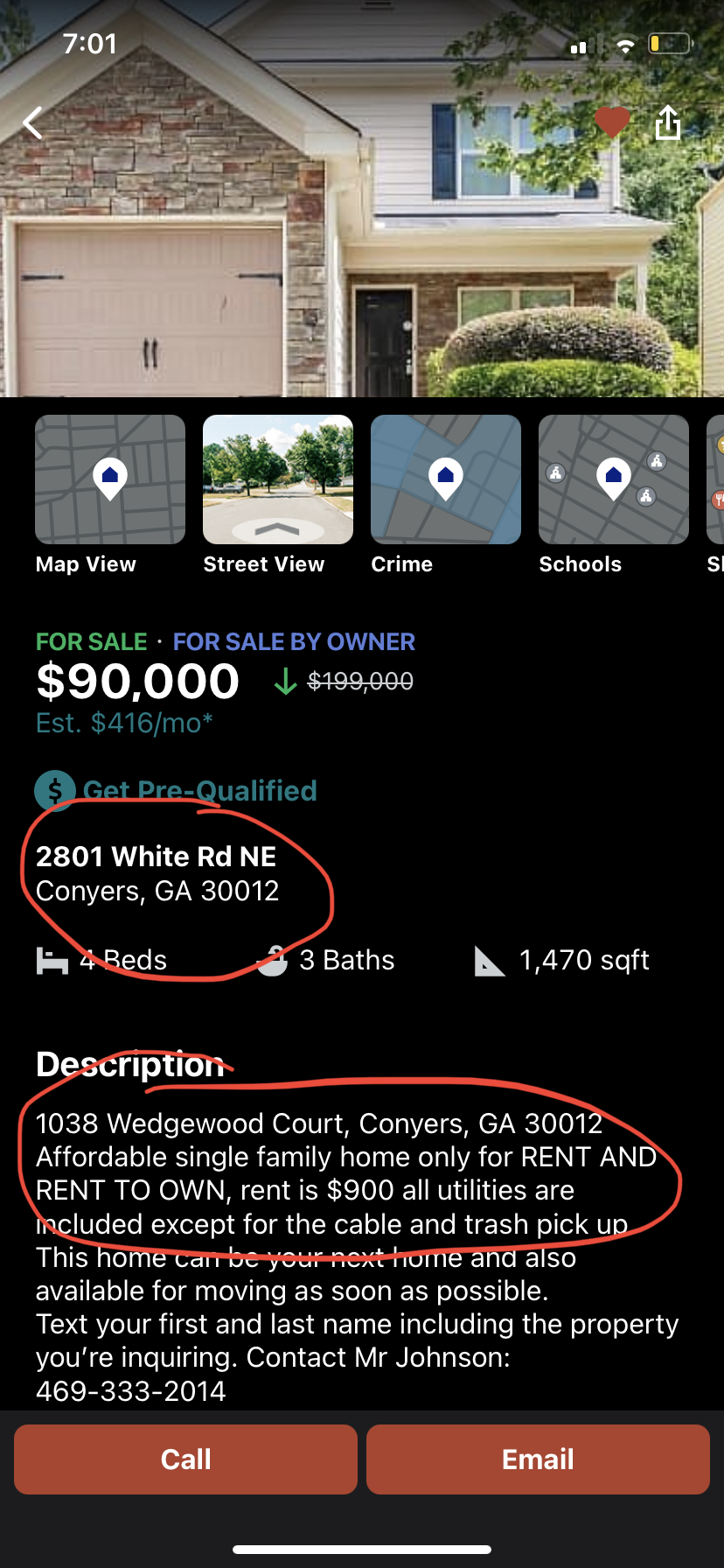**Caption:**

The image prominently features a detailed listing of a property for sale. At the top left corner, "701" is displayed, which may be the property number. Adjacent to this, on the right side, there are four barely visible bars (two white and two gray), a Wi-Fi symbol, and a low battery icon.

To the left, an arrow points leftwards, while on the right side, there are icons of a heart and a square with an upward-pointing arrow.

Below these elements, the image shows different view options and information:
- "Map view" and an associated map image.
- "Street view" and an associated street image.
- "Crime" and an associated map image.
- "Schools" and an associated map image.

In the main section of the listing:
- "FOR SALE" is marked in green and next to a small dot.
- "For Sale by Owner" is in blue, indicating an owner-direct sale.
- The price is prominently displayed in white as $90,000, with a green arrow pointing down from a crossed-out previous price of $199,000.
- In blue, "EST$416-MO" is written with a star next to it, along with a blue circle containing a dollar sign and the text "Get pre-qualified."

The property's address is clearly marked and emphasized with a red circle: 
**2801 White Road NE, Converse, GA 30012**.

Property details include:
- An icon of a bed indicating four bedrooms.
- An icon of a bath (partially covered by a red circle) showing three bathrooms.
- A triangular icon suggesting the property's size of 1,470 square feet.

The description area provides more specific information:
**1038 Wedgwood Court, Converse, GA 30012**:
- Notably marked as an affordable single-family home available for rent or rent-to-own.
- Monthly rent is $900, including all utilities except cable and trash pickup.
- Availability for immediate move-in is emphasized.
- Instructions to text your first and last name along with the property inquiry to Mr. Johnson at 469-333-2014.

At the bottom, two red buttons are visible for "Call" and "Email," facilitating direct contact. The lower section is finished with a white line, possibly for further distinction or navigation purposes.